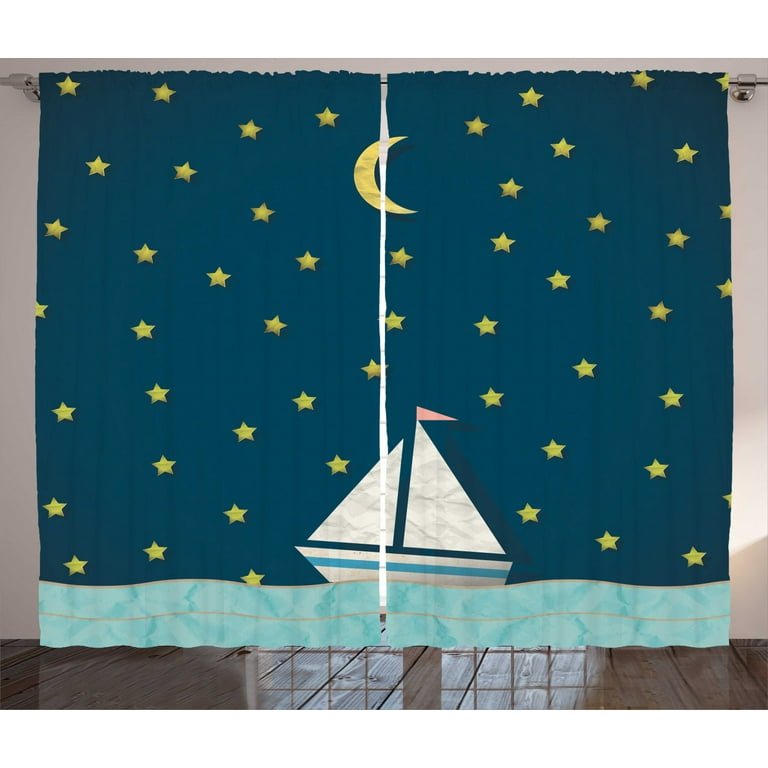This photograph captures a charming decorative curtain set, likely in a child's room. The curtains, hanging neatly from a rod, feature a vividly illustrated scene of a sailboat sailing under a starry night sky. The scene is split across two panels that, when drawn together, form a cohesive image. The lower portion of the curtains showcases light blue, textured waves, simulating a serene ocean. Above, a dark blue sky sparkles with yellow stars and a prominent crescent moon centered at the top. The sailboat, positioned perfectly where the two panels meet, is depicted with white sails and a hull that is white with a light blue stripe along the bottom. At the pinnacle of the sails flutters a delicate pink flag. The wooden floor beneath reflects the sunlight streaming in, adding a touch of warmth to the whimsical night-time seascape.